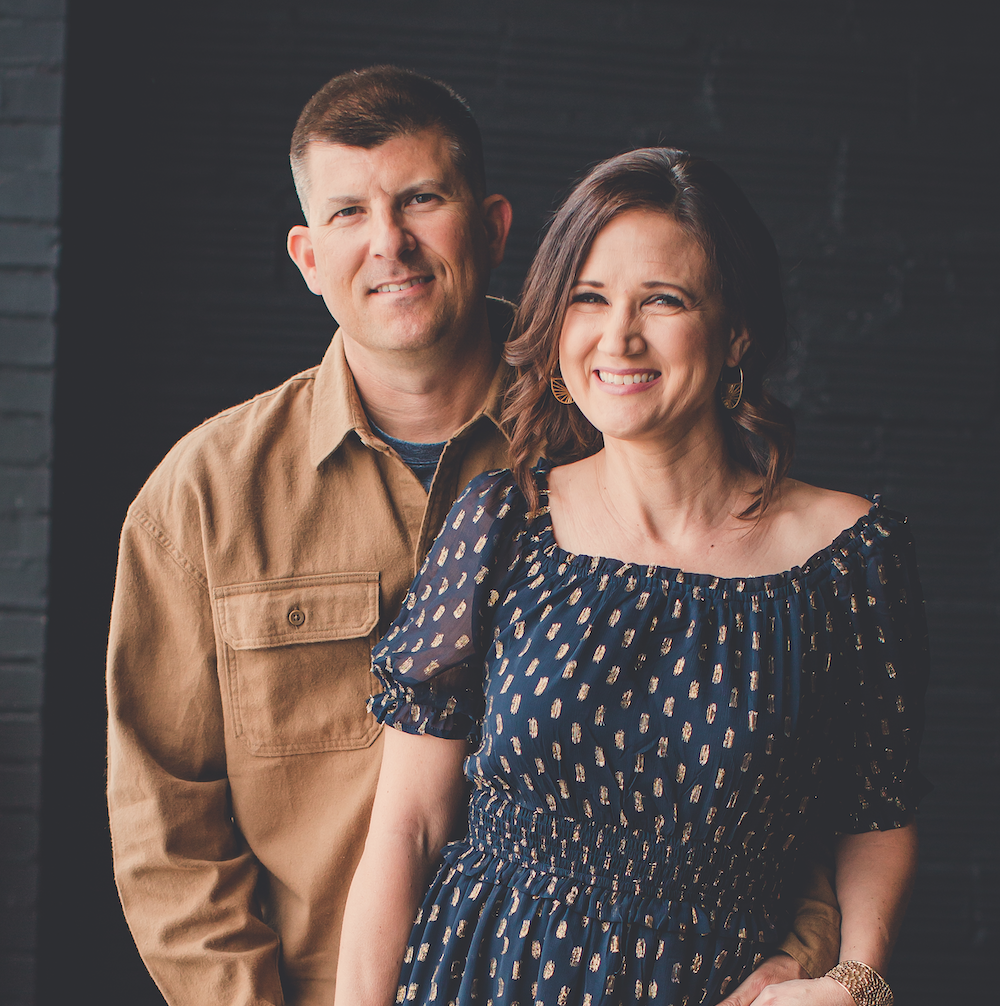This professionally shot photograph features a couple standing closely together against a dark blackish-blue background. The man, who has very short brown hair almost shaved around the ears and a light widow’s peak, is slightly behind the woman. He wears a light brown, long-sleeve shirt with a blue undershirt collar visible. His shirt has a texture that almost gives it a leathery appearance. He has a slight smile on his face and is holding the woman’s left hand with his right. 

The woman, positioned partially in front of the man, has medium-length brown hair that falls just below her shoulders. She is dressed in a navy blue and gold dress adorned with a light beige pattern. Her accessories include dangly earrings and possibly a bracelet or watch, though it's cut off in the image. She is smiling broadly, adding a sense of warmth and connection to the scene. Together, they appear to be in their early 40s.